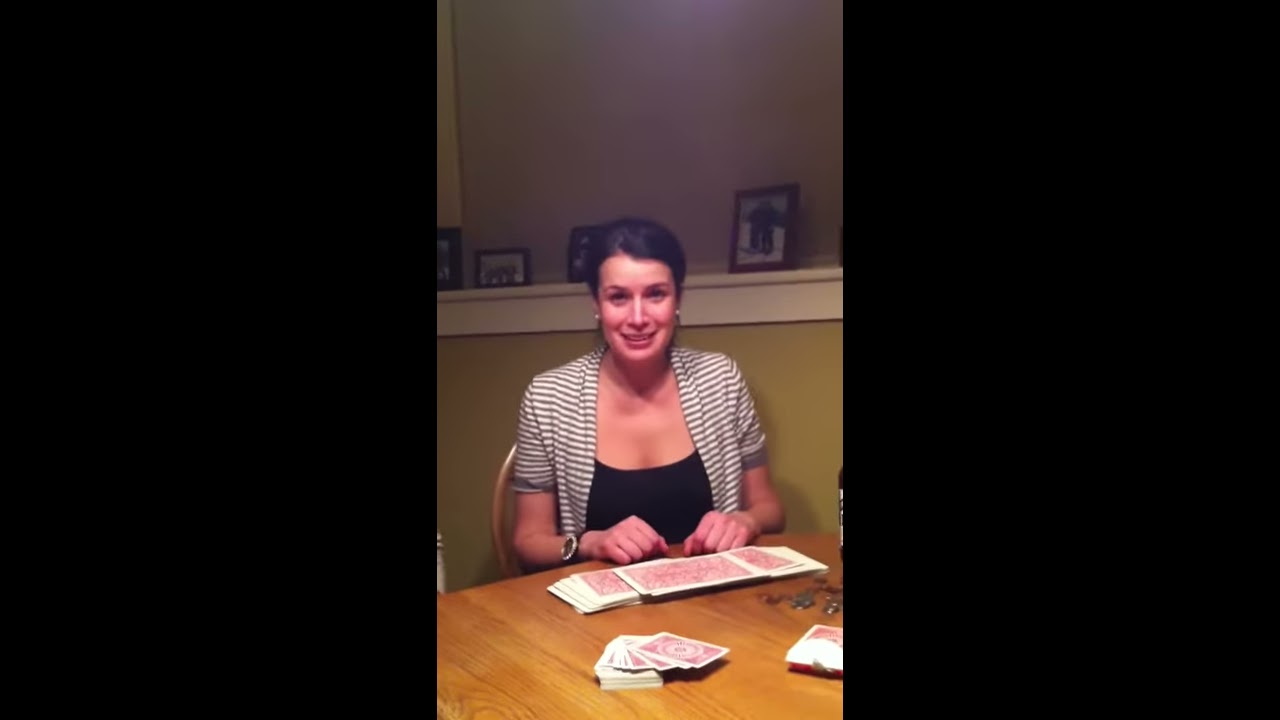This photograph captures a woman, likely in her 30s, seated inside a cozy room. She sits at a round wooden table, vibrant brownish-yellow in color, scattered with red playing cards, including some unusually large ones immediately in front of her. The woman is smiling directly at the camera, her dark brown hair pulled back, revealing small pearl stud earrings. She is dressed in a black camisole or dress, layered with a short-sleeve, horizontally striped cardigan in grey and white tones. A black watch adorns her wrist. In the background, a greenish-grey wall hosts a white shelf with framed photographs, creating a homely ambiance. Additional details include faint overhead lighting and a barely-visible can of beer on the right edge of the frame, along with black vertical strips flanking either side of the image.